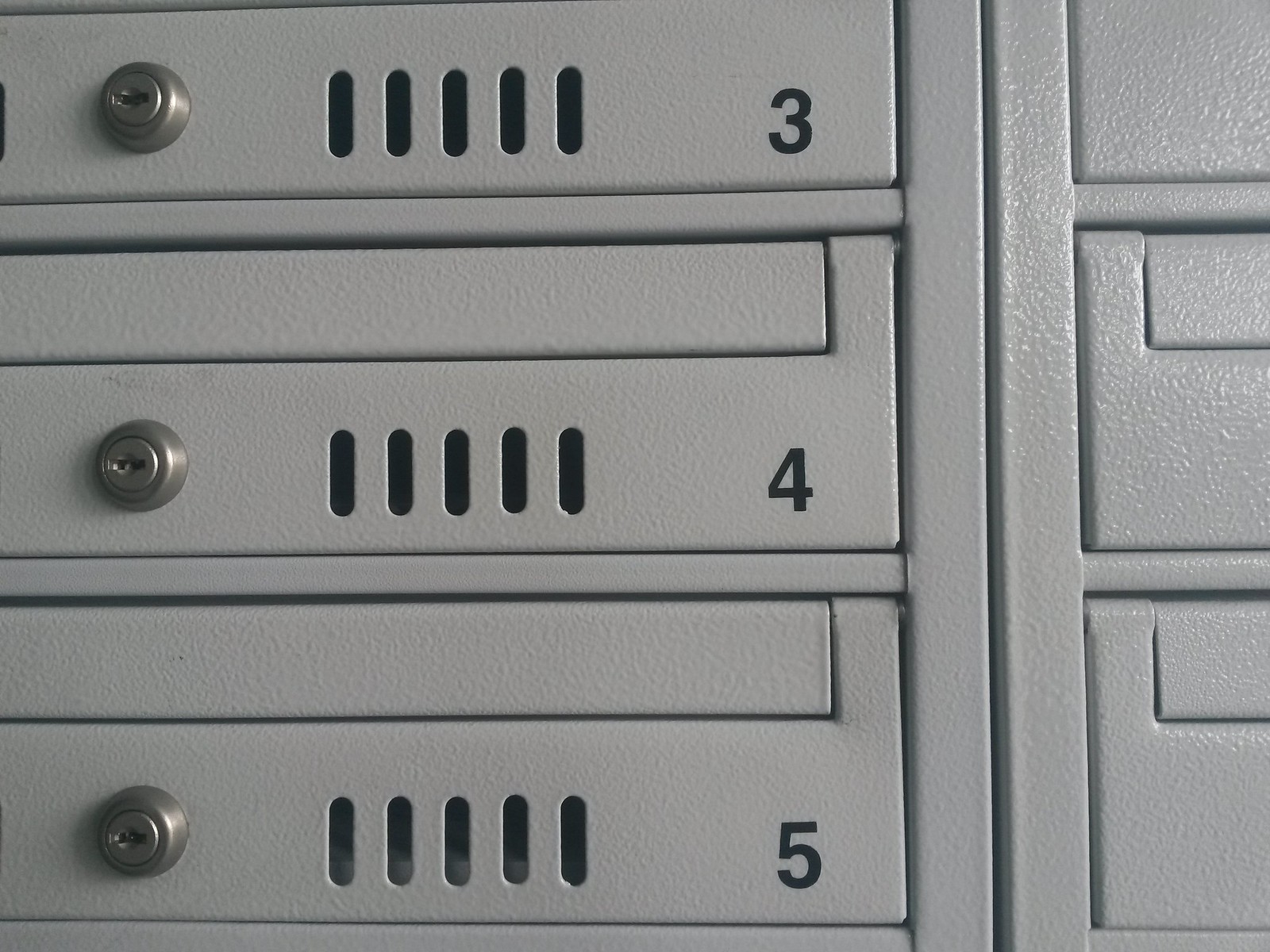The image depicts a close-up view of a series of small metal lockers, possibly used as secure drop boxes or lockboxes. Each locker is painted in a light gray color with a slight greenish khaki tint, reminiscent of a camouflage palette. The focus is on a vertical stack of three lockers, numbered sequentially from top to bottom as three, four, and five. Each locker features a circular keyhole and a set of five vertical ventilation slats positioned between the keyhole and the number. Although additional lockers can be seen on the right side of the image, their details, including numbers, are not visible. Horizontal beams also intersect the lockers, adding to the structural framing of the image. The lockers may be part of a larger secure storage system, typically found in environments like banks or delivery drop-off points.